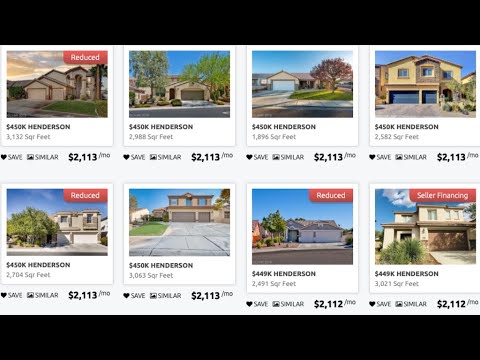The horizontally rectangular image is a detailed screenshot from a real estate listing site, characterized by black horizontal banners at the top and bottom. Inside, there are two rows with four listings each, showcasing exterior images of homes. All properties are situated in Henderson (exact location unspecified).

The top left, bottom left, and the third listing in the bottom row are marked as "Reduced," indicating lowered prices. The fourth listing in the bottom row is marked as "Seller Financing."

Most homes are listed at $450,000, with the exception of the last two listings on the bottom row, listed at $449,000. Monthly payments for the majority of the homes are $2,113, while the last two bottom right listings are $2,012 per month.